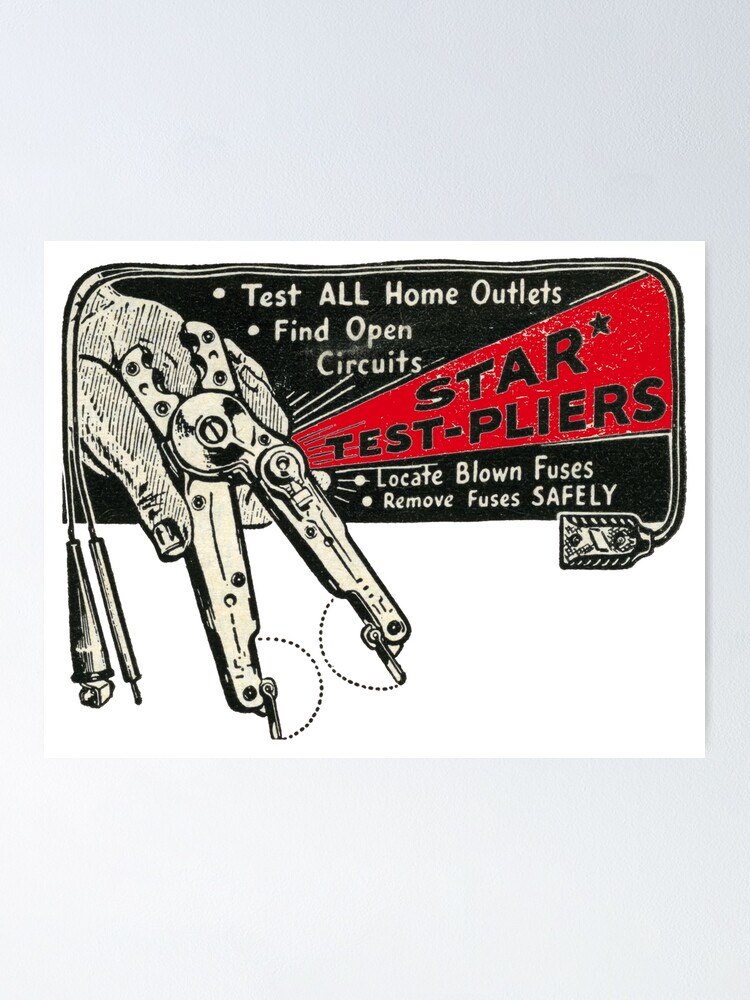In the center of this image, there's a detailed drawing of a white piece of paper featuring an advertisement for a set of test pliers used by electricians. The focal point is a meticulously illustrated hand in the top left corner, shaded with brownish tones, gripping a pair of electrical testing pliers. The pliers appear brownish like the hand and create two incisions on the paper, marked by dotted lines. The advertisement blends vivid colors and text. At the top right, in black and red text, it reads "Test all home outlets" and "Find open circuits." Below that, there's a red background with "Star test pliers" prominently displayed. Further down, it highlights the instructions "Locate blown fuses" and "Remove fuses safely." This illustrative and instructive ad serves as a reminder for electricians on how to properly test electrical circuits, emphasizing the functionality and reliability of the Star test pliers.